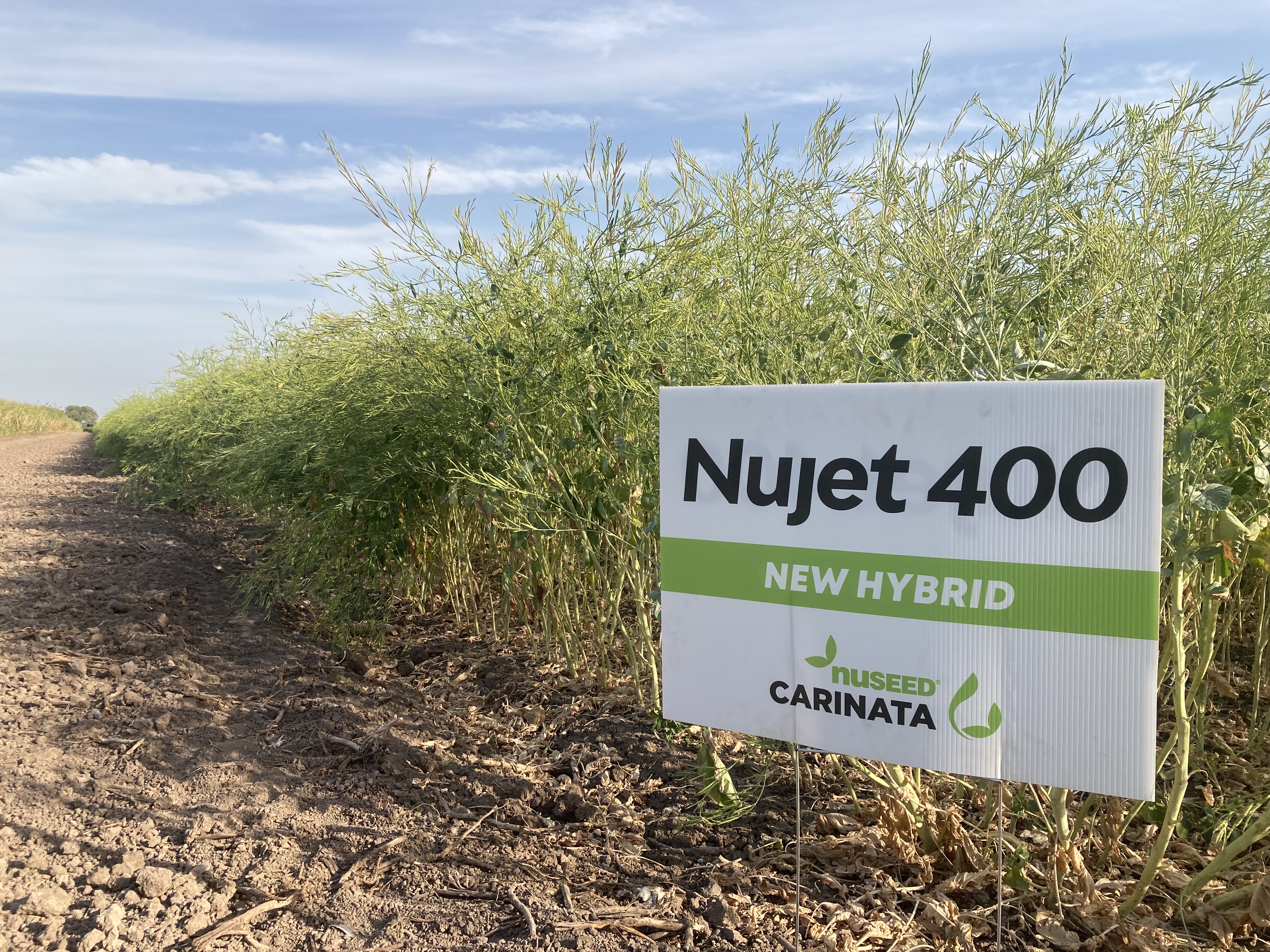This color photograph captures a detailed scene of an agricultural crop plot on a bright day, marked by a vivid blue sky with scattered clouds. The focal point of the image is a white sign with black and green text, mounted on two metal poles. The top of the sign reads "NUJET 400" in bold black letters, followed by a green banner in the middle containing the text "New Hybrid" in white. At the bottom of the sign, "NUSEED" is written in green, next to the bold black text "CARINATA," flanked by stylized illustrations of green leaves. In front of the sign lies a row of bushy plants, about two feet tall, with fine, thin leaves and tan-green stems, planted in straight lines within the clear, brown dirt that stretches to the left. To the right, the dense green crops contribute to the lush agricultural setting.